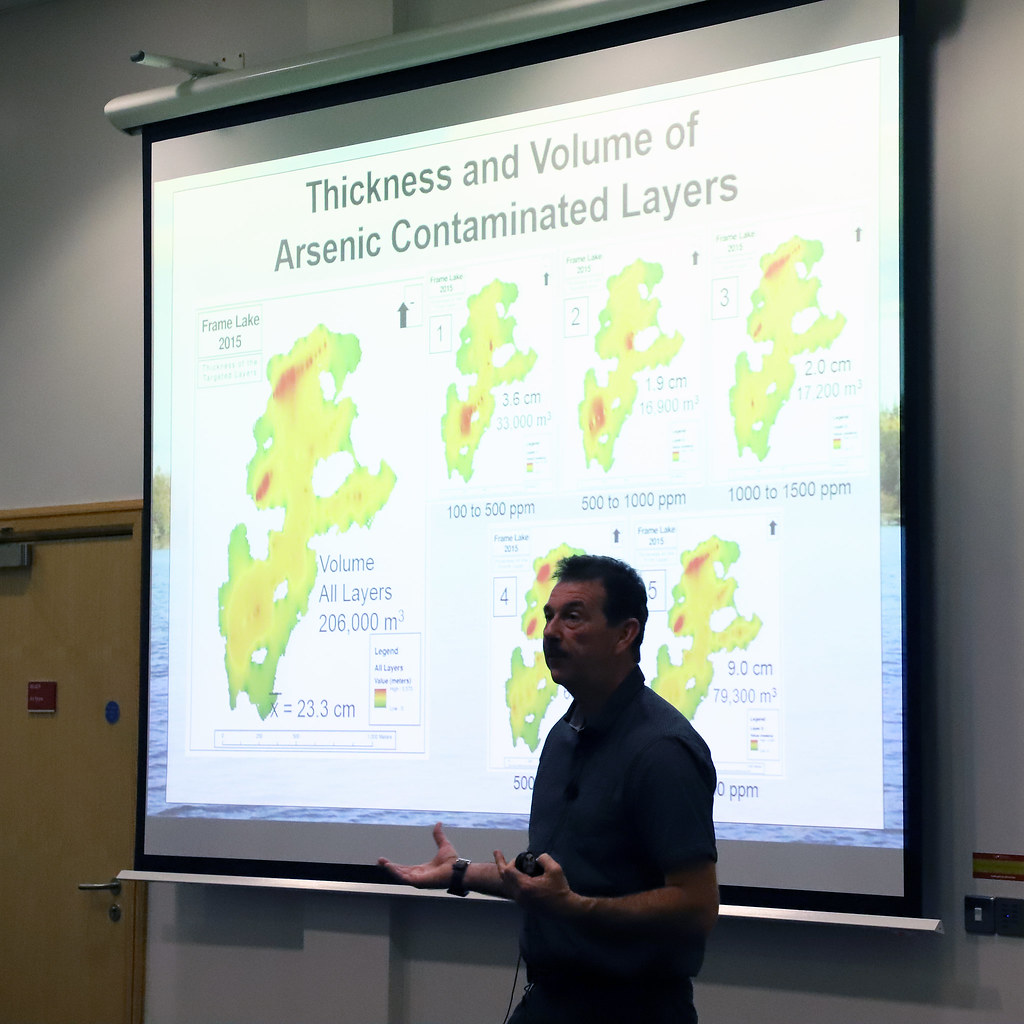The image captures an engaging lecture in a typical college classroom, characterized by tall white walls and a wooden door on the bottom left side. At the center of the scene is an older man with black hair and a mustache, dressed semi-professionally in a dark short-sleeved shirt. He stands with a microphone in hand, his serious gaze directed to the left, indicating he is in the midst of lecturing. Behind him, a projection screen displays a detailed PowerPoint presentation titled "Thickness and Volume of Arsenic-Contaminated Layers" in black text. The screen showcases multiple thermal-like images displaying green, yellow, and red layers, illustrating the contamination levels in Frame Lake over various years. These images are organized with maps labeled from 1 to 5, indicating the parts per million (PPM) of arsenic and the volume in cubic meters (m³) for each layer. The presentation includes a wealth of data, emphasizing the degree of contamination and its progression.